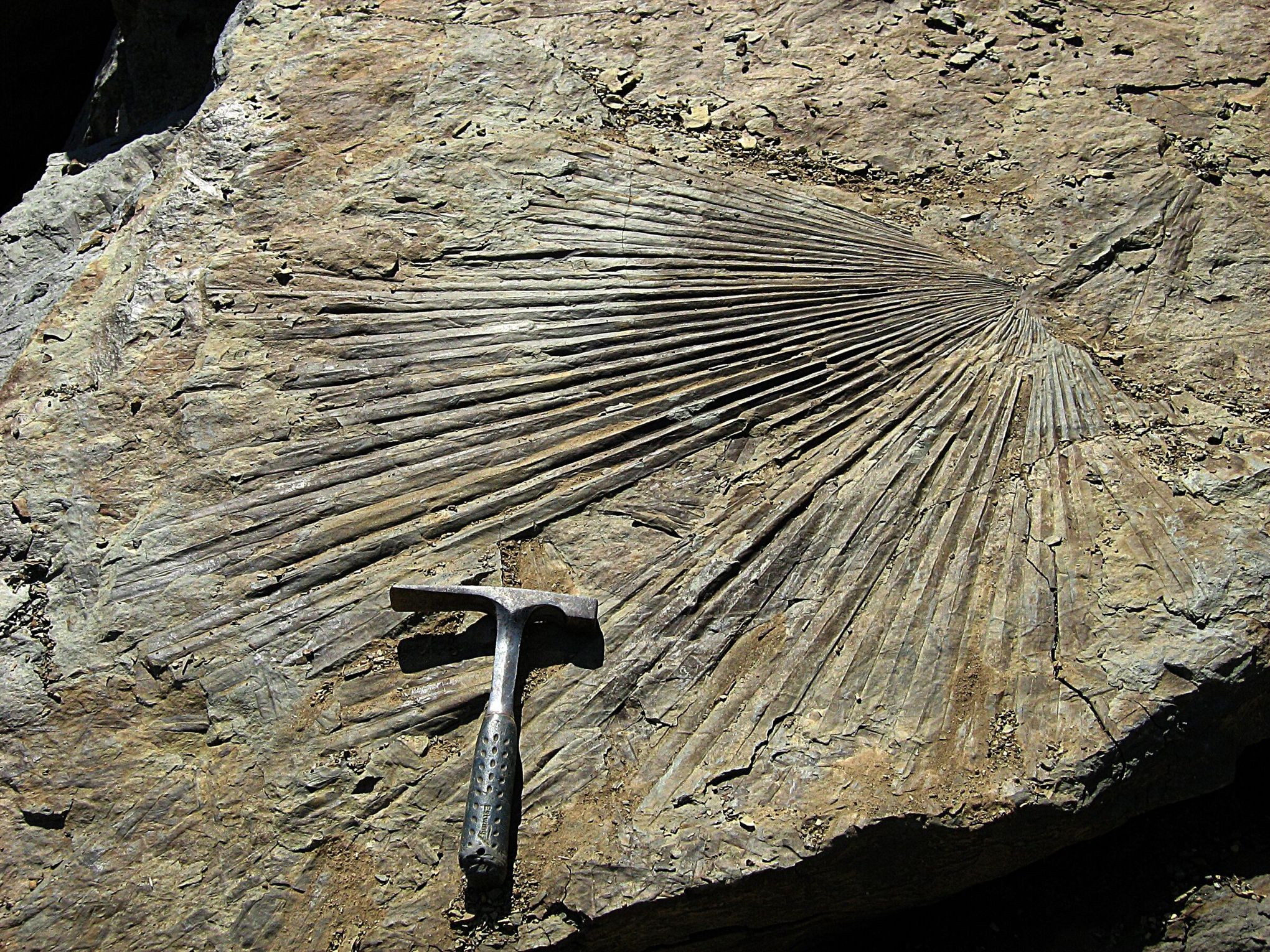The image shows a sunlit scene taken from above, featuring a large, flat, jagged-edged rock that occupies the majority of the frame. The rock is a mix of gray and brown shades. It prominently displays a fossil, likely of a fan palm or frond, easily recognizable by its zigzag ridges and a stalk pointing toward the top right corner of the image. In the bottom third of the image rests a hammer, used for excavation, with a black handle and a head featuring both a flat square and an angled chisel side. The photograph is brightly lit, suggesting it was taken around high noon, with only the top left and bottom right corners shrouded in darkness.